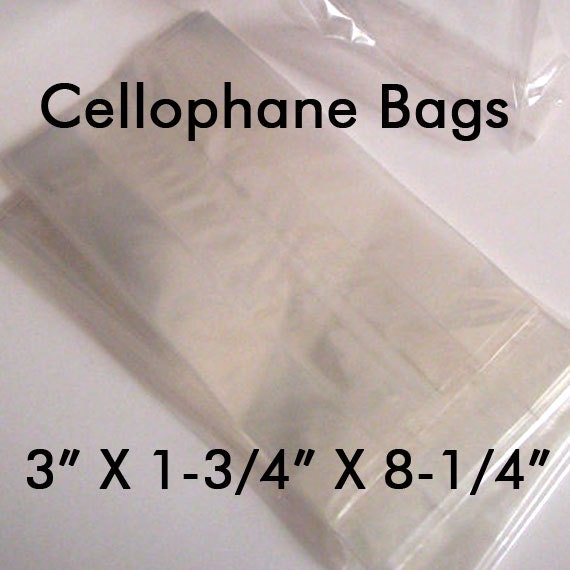This image features a stack of rectangular cellophane bags displayed diagonally across a white table or background, extending from the top left corner to the bottom right corner. In the top portion of the image, large black letters prominently spell out "cellophane bags." Below the bags, centered at the bottom of the image, the dimensions are clearly marked in black text as "3 inches by 1 and 3/4 inches by 8 and 1/4 inches." One bag in the upper right-hand corner appears to be separate from the stack, suggesting it may be partially open. The overall background is a light grayish-white, adding a clean and minimalist aesthetic to the presentation. The bags themselves are transparent, and inside one of them, items that resemble folded napkins or tissues can be seen.